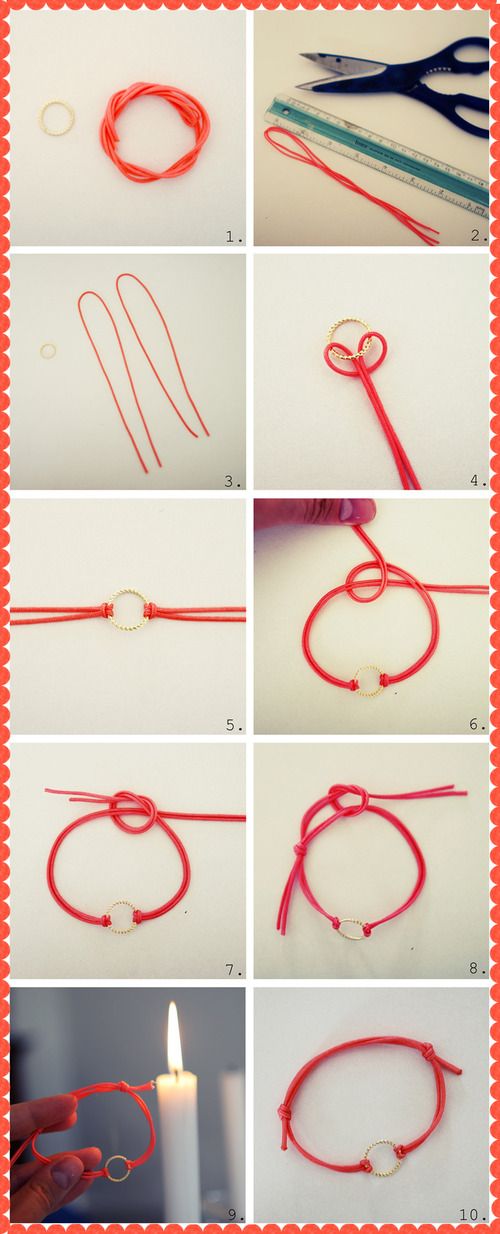The image features a step-by-step guide on how to create a bracelet using red and pink yarn and a circular piece of jewelry, framed within a red-bordered box organized into ten panels. Starting from the top left, Panel 1 shows the necessary materials: red and pink yarn, a circular piece of jewelry, black-handled scissors, a blue-and-clear ruler, and a small piece of red lace. Panel 2 and 3 show two U-shaped loops of the yarn, while Panel 4 depicts the yarn loops threaded through the circular jewelry piece. Panel 5 demonstrates the initial formation of the bracelet with the circular piece centralizing the design. By Panel 6, a finger is seen tying the yarn into a knot, progressing into Panels 7 and 8 where the knot is gradually tightened, ensuring the jewelry stays secure. Panel 9 introduces a candle, illustrating the process of sealing the knot by melting the ends with a candle's flame, seen in a person's hand. Finally, Panel 10 showcases the completed bracelet, fully assembled and ready for wear. Each step is clearly labeled from 1 through 10, laid out in a grid of white squares with the instructional details visually and descriptively presented against mostly white backgrounds, except for the candle process on a gray background. The entire setup appears to be indoors, focusing on providing a detailed, creative guide in an arts and crafts style.